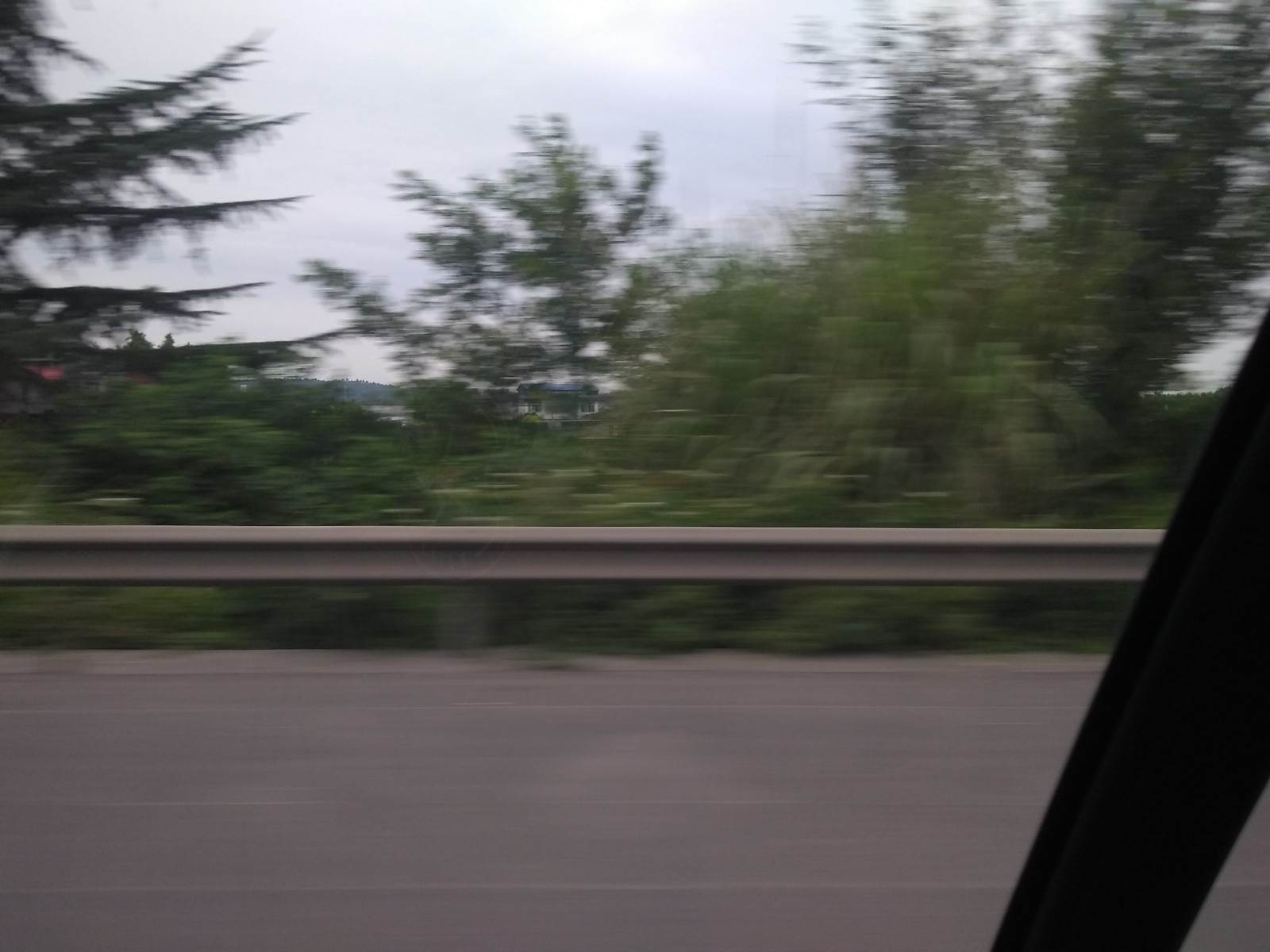A blurry photograph captures the scene from a moving car window, exuding a sense of speed and movement. The unfocused image showcases the gray pavement rushing past, and part of the car’s window pillar intrudes on the right side of the frame. A horizontal gray railing runs across the middle of the picture, acting as a boundary between the roadside and the landscape beyond. In the blurred background beyond the railing, a mixture of trees and thick green foliage is visible, with a distinct pine tree standing out to the left. The remaining trees form a vague, blended mass of greenery, merging into a distant view of lush vegetation under a clear blue sky.